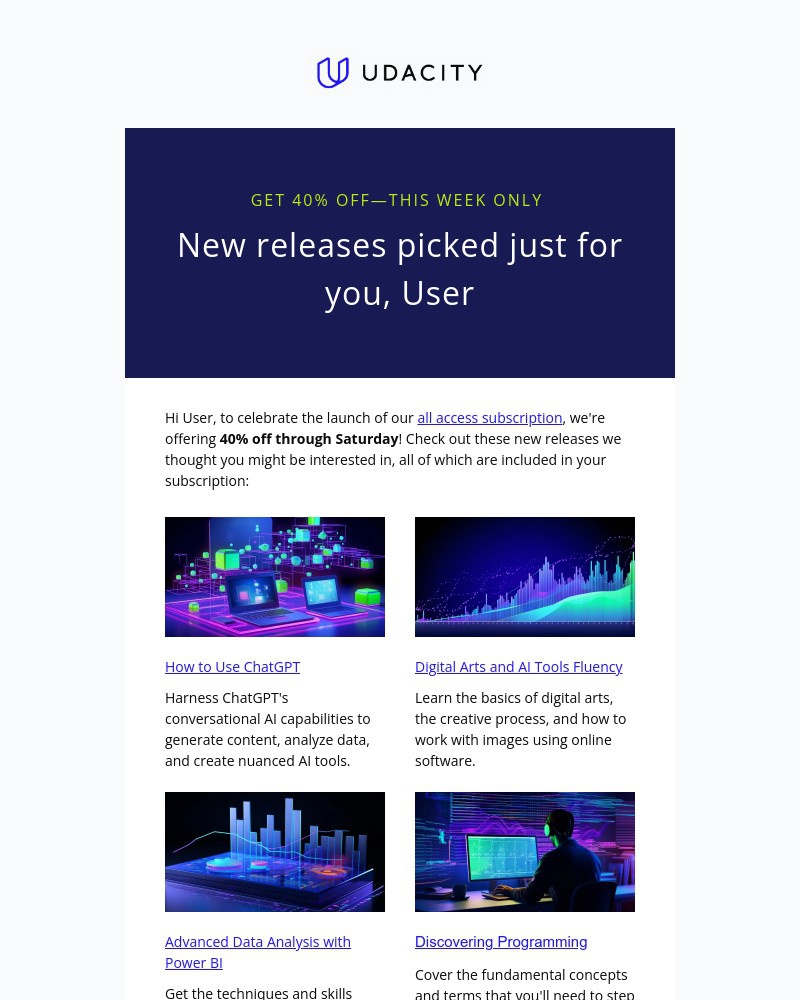This is a detailed digital photograph, possibly a computerized snapshot of a webpage for Udacity, prominently displayed in small capital black letters alongside a distinctive 3D blue "U" logo. The highlighted promotion announces a 40% discount available this week only to celebrate the launch of their all-access subscription. The page greets with "Hi user," and invites exploration of new releases tailored for the user, all included in the subscription. Featured courses include 'How to Use Chat GPT,' 'Digital Arts and AI Tools Fluency,' 'Advanced Data Analysis with Power BI,' and 'Discovering Programming,' which covers fundamental concepts and terminology. The page is well-lit with a glow visible on a computer monitor in the bottom right-hand corner.